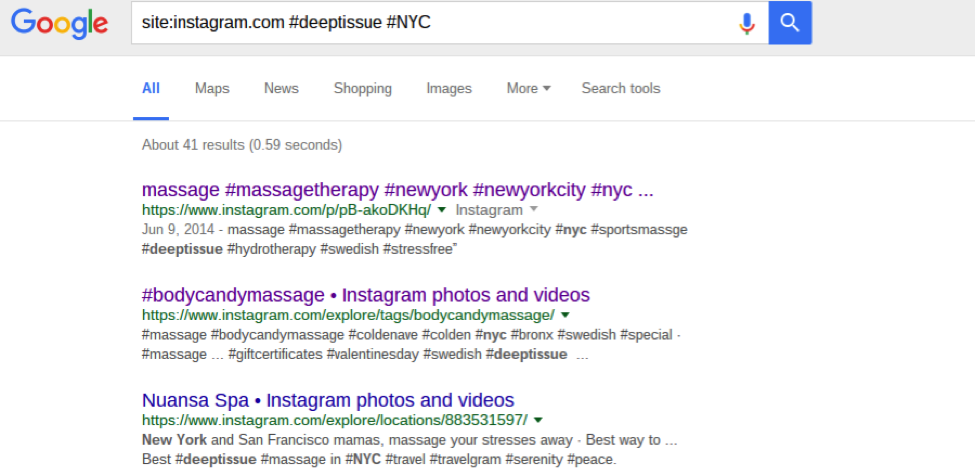The image depicts a Google search query conducted with the specific aim of finding Instagram posts related to "deep tissue" massage in "New York City." The search string entered was site:instagram.com "deep tissue" "New York City," and the results were generated in 59 seconds, with a total of 49 comments found. 

The top result is for an Instagram post tagged with terms such as massage, massage therapy, New York, New York City, and NYC, making it closely aligned with the search criteria and highlighting deep tissue services. The second result is for "Body Candy Massage," also located in New York City and offering deep tissue treatments, clearly stated on its Instagram profile. The third result features UANSA Spa's Instagram photos and videos, which likewise offers deep tissue massage services in New York.

At the top of the search results page, the iconic Google logo is visible on the left, rendered in its characteristic colorful style. Adjacent to this logo is a microphone icon, indicating the option to perform a voice search. Next to the search bar itself is a blue button labeled "Google Search," allowing users to initiate the search once the query is typed in. Each search result appears as a clickable hyperlink, enabling users to directly navigate to the relevant Instagram posts.